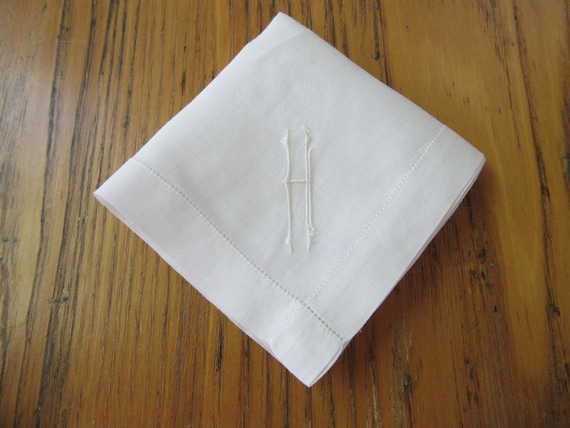In the image, we see a folded white linen napkin placed on a horizontally oriented, orangey-brown wooden surface with darker grain creases. The napkin, folded into a square and positioned diagonally to resemble a diamond, showcases an embroidered pattern in its center that resembles an 'H'. This 'H' is formed by two vertical lines connected by a shorter horizontal line in the middle, with additional detailing at the ends of these lines. The seams of the folded napkin run from the lower left to the bottom right corners, with a slight crinkle visible at the top. The napkin occupies much of the vertical space in the frame, leaving more visible table surface on the sides, and a slight glare appears on the left side of the table. The main colors in the image are white, brown, and black, with no text present.